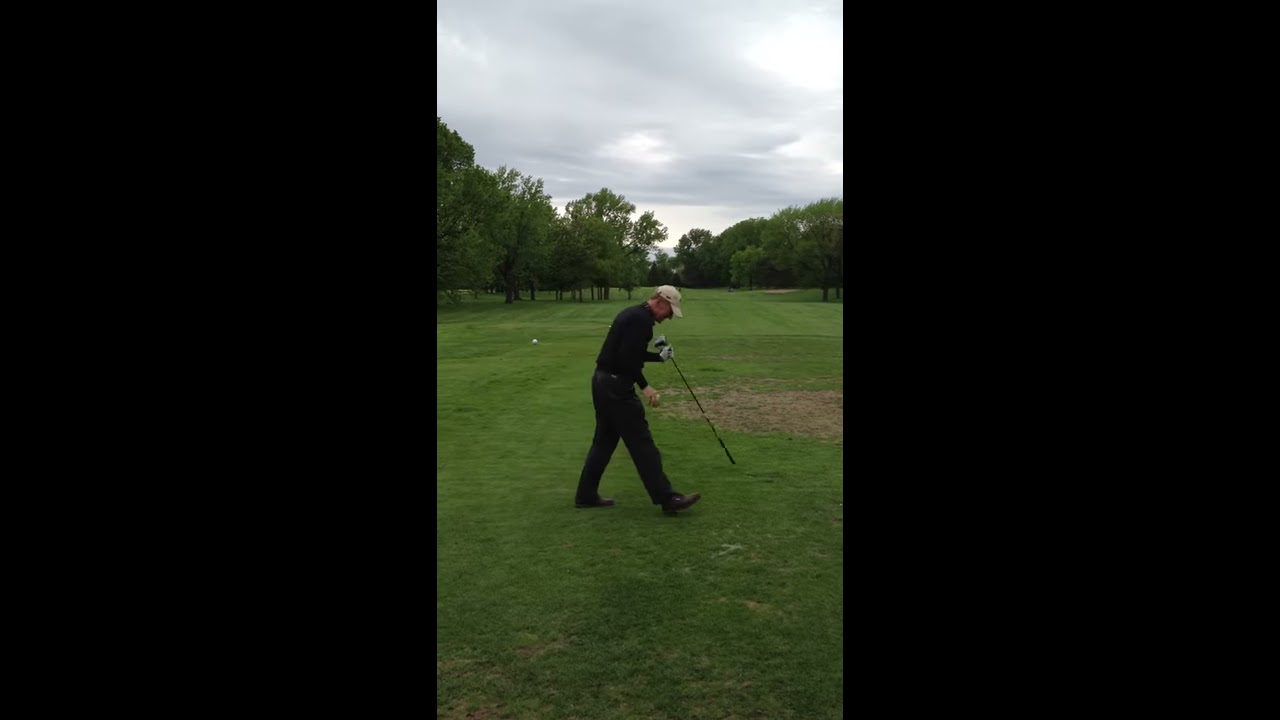In the image, a man is captured on what appears to be a golf course. The scene features a vibrant green expanse with some bald patches of grass, particularly a noticeable brown patch toward the center. The golfer, mid-step and slightly bent over, seems to be preparing to either place or pick up a golf ball or tee. He is wearing a beige or khaki hat, a black long-sleeved shirt, long black pants, and black shoes. A white golf glove is visible on his left hand, which holds a golf club upside down with the club's head in his hand and the handle pointing towards the ground. 

In the background, tall green trees line the course, adding depth to the scene. The sky is overcast and gray, suggesting an imminent storm or rain, providing a hazy and somber backdrop. There is a small white object in the distance on the ground, possibly part of the golf course equipment. The image itself is cropped with black rectangles on either side, directing focus on the central scene.